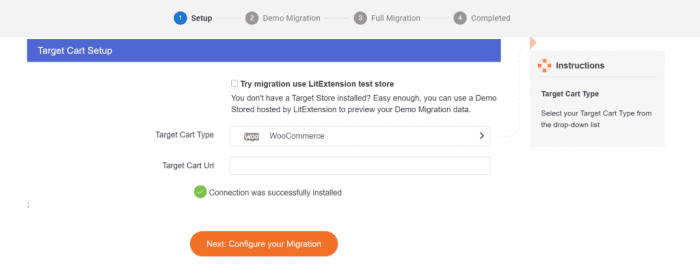The image is a screenshot or mock-up, likely being used as a slide in a PowerPoint presentation, depicting a step-by-step process for configuring a migration. It has a primarily white background, with central elements organized to guide the viewer through the setup.

At the top of the image, there are four circles labeled "1, 2, 3, 4." The first circle is highlighted in blue, showing the current step labeled "Setup" in bold black text, while the other three circles are gray and labeled "Demo Migration," "Full Migration," and "Completed."

Below the circles, a blue banner with white text reads "Target Cart Setup." Underneath this banner, several options are presented. The first option is "Target Cart Type," with "WooCommerce" selected from a dropdown menu. There's an arrow indicating further options available in the dropdown. The next option is "Target Cart URL," which is a blank text entry field.

A green checkmark and the message "Connection was successfully installed" indicate a successful connection. Between the options and the blue banner, a checkbox labeled "Try migration to use LIT extension test store" is shown.

To the right of these elements, an "Instructions" section, marked by an icon with four red dots, draws attention. This section provides further guidance: "Target cart type: Select your target cart type from the drop-down list."

The image appears to be either a cropped screenshot or a designed mock-up, used to illustrate the migration setup process in an instructional or presentation context.